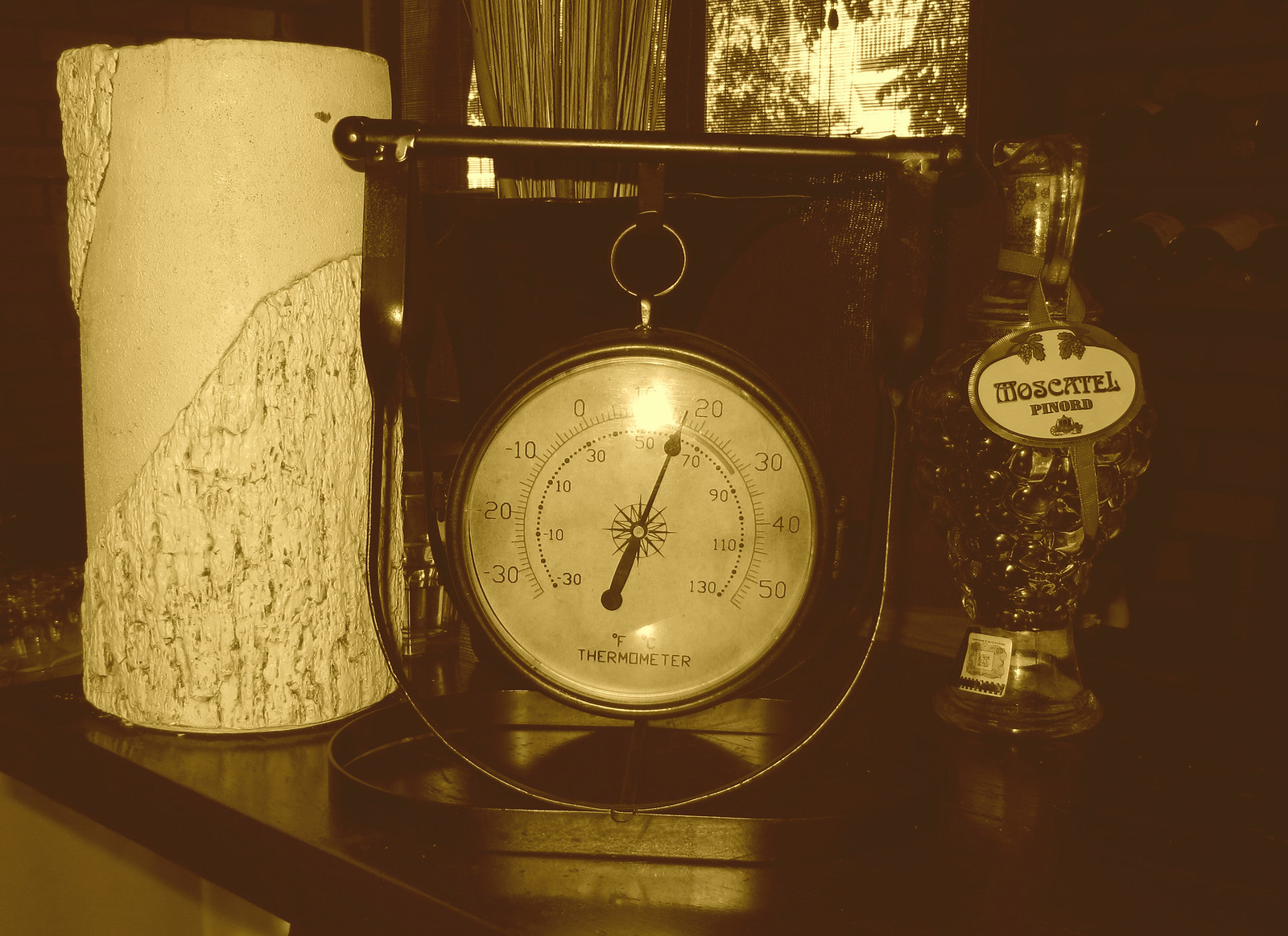In the image, a thermometer with a distinctive yellow filter dominates the foreground, prominently displaying a face reminiscent of a stopwatch. The thermometer's scale ranges from -30 to 50 degrees, marked in both Fahrenheit and Celsius, with a central needle and decorative stars encircling the dial. On the left-hand side, a large, cylindrical candle with a rugged, rock-like texture stands out, showcasing its intricate ridges, edges, and cracks. The scene is set on a countertop with a sleek black surface, contrasting against a white wall in the background. In the distance, sheer curtains partially drawn over blinds reveal a hint of leaves outside. To the right, a clear bottle filled with what appears to be marbles and labeled "Moscatel Pinot" provides an intriguing detail. The overall atmosphere is a blend of functional simplicity and subtle complexity.